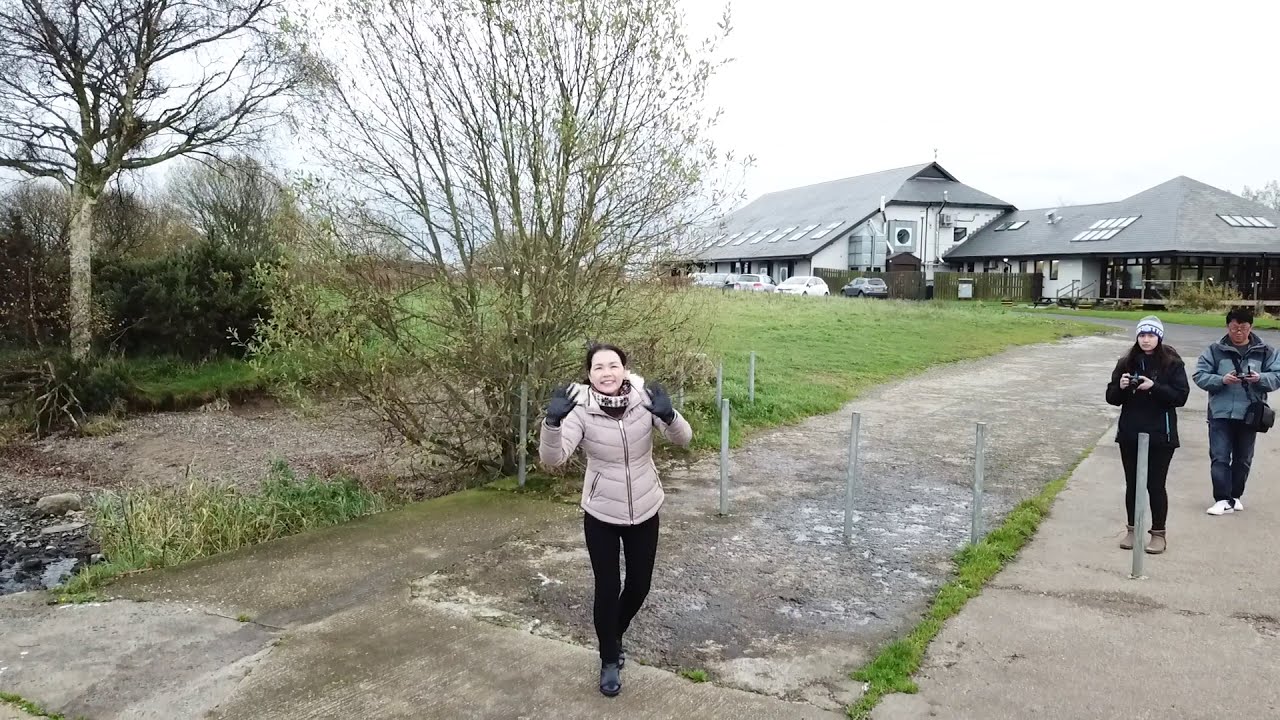In this photograph, taken in an outdoor setting during daylight with abundant natural light, a woman stands in the center, looking directly at the viewers with a joyful smile on her face. She is wearing a cream-colored jacket, a beige scarf, black pants, and black boots, along with black gloves, which she is holding up as if showing or displaying something. Her light skin and black hair are illuminated by the natural light.

To the right of the woman, further back along a concrete pathway, two figures, one male and one female, are seen holding cameras, seemingly waiting to take their own picture. The pathway is bordered on the left by a grassy area with a few trees, which appear bare, suggesting early spring with hints of lingering cold.

In the background, there is a low building, perhaps a large home, outfitted with solar panels on its roof. Various parked cars can be spotted near this building, adding to the comprehensive view of the scene. The sky above is entirely overcast, casting a uniform white light over the entire setting.